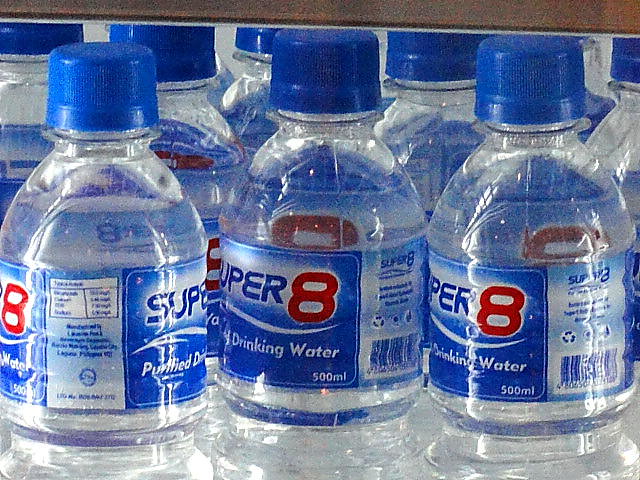This close-up photograph captures an array of 500 milliliter Super 8 Purified Drinking Water bottles, likely situated in a refrigeration case, possibly in a convenience store. The scene is filled with the top sections of approximately ten clear plastic bottles, each crowned with a blue cap. The labels, predominantly blue with a darker blue banner, prominently feature the brand name "Super 8" with the numeral 8 in red and "Purified Drinking Water" in white. The three bottles in the foreground are fully visible, though some labels are turned to the side, obstructing the full text. Behind these, additional bottles are aligned, with their clear nature and reflective surface beneath hinting at a well-lit, polished refrigerator environment.